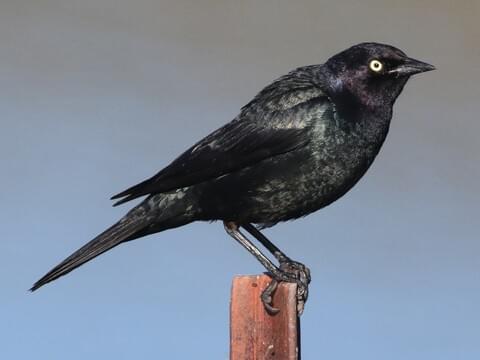The photograph features a small, jet-black bird, likely a blackbird or magpie, perched atop a light brown wooden post. Captured in a right-facing side profile, the bird's long tail feathers extend towards the bottom left corner of the image, while its head is positioned in the top right corner. The bird's short beak, large vivid yellow eye with a black pupil, and black talons gripping the post are prominently visible. The background is a gradient of indistinct bluish-gray hues, transitioning from a lighter blue at the bottom to a darker shade of blue and gray towards the top, which emphasizes the bird's dark silhouette. The wings of the bird are tucked neatly against its body, while its thin black legs are positioned firmly on the wooden post, suggesting a secure perch.